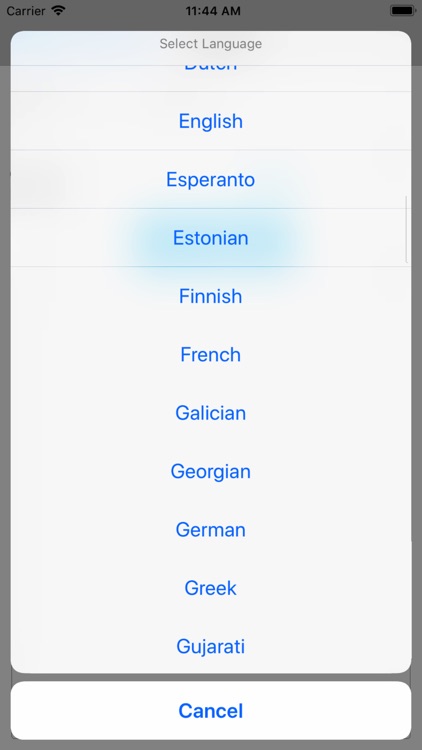A screenshot of a cell phone screen showing a language selection menu outlined in grey. At the very top, there is a dark grey bar indicating it is 11:44 AM, with a Wi-Fi signal icon, the word "carrier," and a fully black-colored battery symbol. Below this, a large grey rectangle features a horizontally-aligned list of language options displayed in blue text: English, Esperanto, Estonian (highlighted in light blue), Finnish, French, Galician, Georgian, German, Greek, and Gujarati (spelt G-U-J-A-R-A-T-I). The top grey bar inside the rectangle reads "Select Image" in grey text. At the bottom of the screen, in a separate small grey rectangle, the word "Cancel" is displayed. There are no additional details or text visible on the screen.